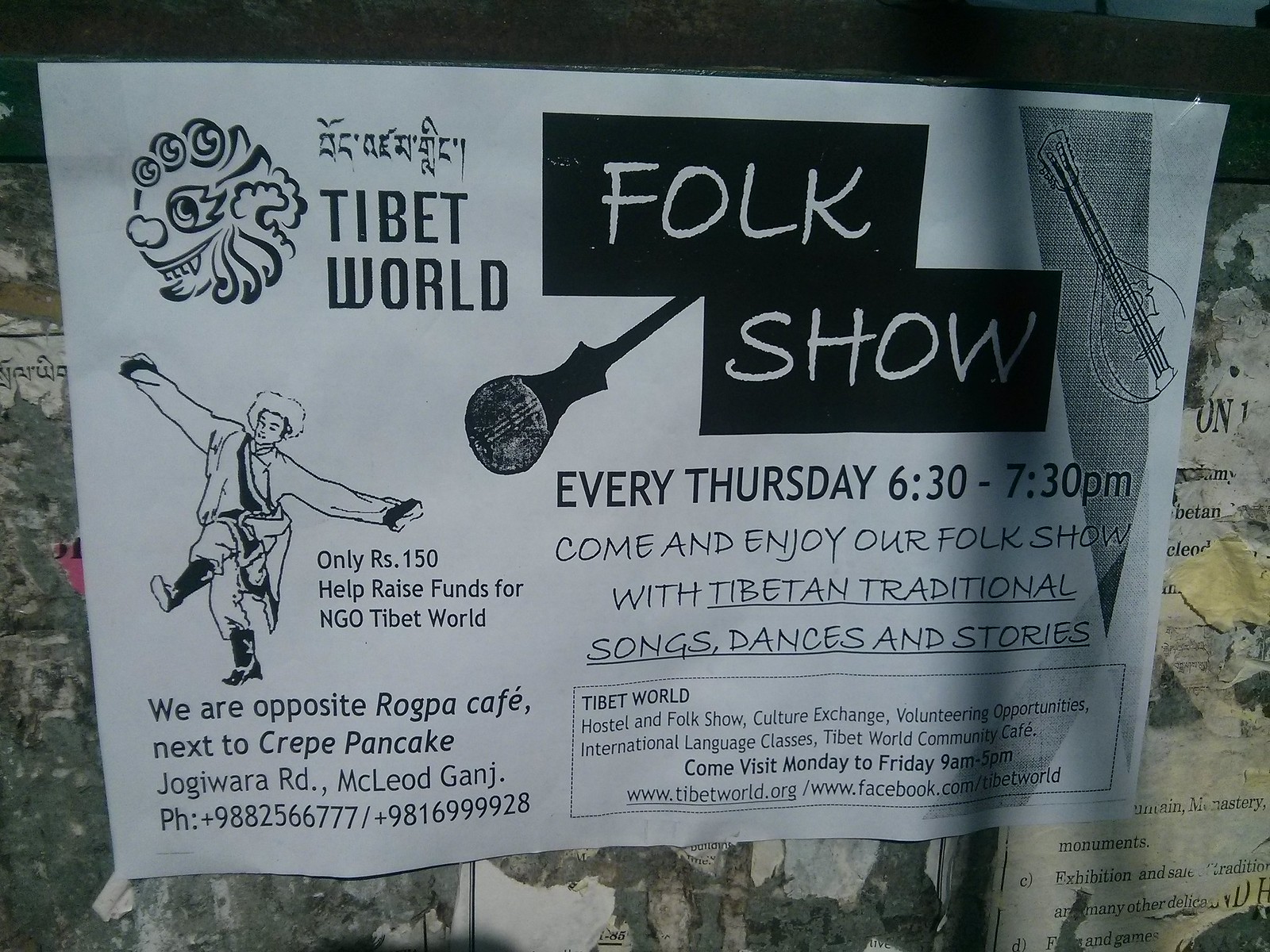The image is of a black and white poster attached to a grey, cement wall covered with the remnants of various other torn-off posters. This rectangular flyer is an advertisement for the "Tibet World Folk Show," which takes place every Thursday from 6:30 to 7:30 PM. It invites viewers to enjoy an array of Tibetan traditional songs, dances, and stories. The top of the poster prominently features the event name "Tibet World Folk Show," with a dragon drawing in the upper left corner and an outlined guitar in the upper right. Additionally, there is an image of a man in traditional Tibetan clothing dancing on the left side of the flyer. Below the main text, the poster mentions that entry costs RS-150 and the proceeds will help raise funds for the NGO Tibet World. It provides the location as opposite Rapa Saw Cafe, next to Crepe Pancake on Jawaga Road, McLeod Ganj. Contact information includes two phone numbers: +98 825-667-7777 and +98 169-999-9928. The poster also features a peculiar face icon, possibly a clown, reflecting an element of Tibetan cultural design.